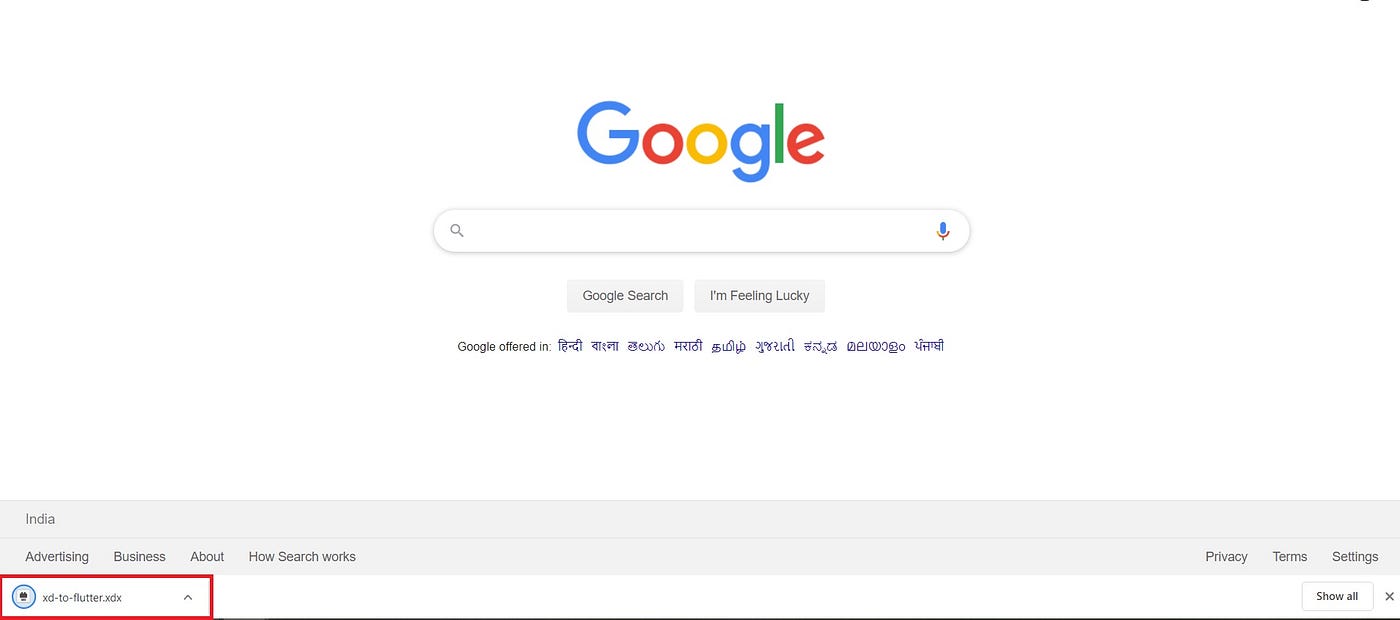The homepage of Google.com is displayed prominently, featuring the iconic "Google" logo, with each letter in a distinct color: the capital "G" in blue, the first "o" in red, the second "o" in yellow, the lowercase "g" in blue, the "l" in green, and the "e" in red. Below the logo is a white search bar, accompanied by a magnifying glass icon on the left, and a microphone icon on the right for voice searches. Beneath the search bar are two buttons: "Google Search" and "I'm Feeling Lucky."

Further down, the page indicates that Google offers its services in various languages, identifiable by what appear to be Indian script characters. The bottom section of the page is a light gray footer featuring the word "India." Below this, there is a series of links including "Advertising," "Business," "About," "How Search Works," "Privacy," "Terms," and "Settings." Additionally, an outlined red box highlights a downloaded file named "xd-to-flutter.xdx," indicating a recent download on the computer.